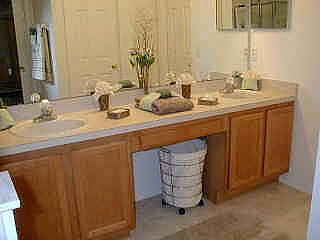The image captures an intimate view of a bathroom taken indoors with a regular camera. The focal point is the bathroom counter, which features a single sink with a solitary spigot. Below the sink, there are four separate cupboards, flanking a slim central drawer. Adjacent to this is a compartment that houses a trash can or hamper. A wire basket organizer sits on the floor, distinguishable by its four black wheels. 

The countertop is adorned with decorative items including a neatly laid-out towel, a vase filled with flowers, and two additional cups that also contain floral arrangements. Positioned on the linoleum floor is a small rug, adding a touch of coziness to the space.

On the left side of the image, a white cabinet is partially visible, while the reflection in the large mirror on the back wall reveals a towel hanging from a towel rack. To the right, a panel door closet with four sections stands against the wall, its white panels complementing the overall aesthetic. A small picture frame is hung on the right wall, contributing to the room's decor.